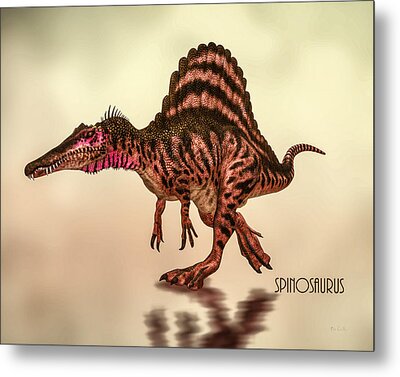The image is a detailed, colorful illustration of a Spinosaurus, presented against a blend of beige, gray, and pink background. The dinosaur takes the central position in this artistic, magazine or book cover-like composition. The Spinosaurus has a distinctive alligator-shaped head with white teeth, and a magenta-colored chin. Its eyes are pink, and it features pink and brown hues around its head and neck, adorned with small spikes. The creature's back is bumpy and topped with a large, round, curvy spine that extends into a substantial hump, eventually tapering into a tail on the right side. The body has a brown base with black spots, while its short arms with three claws dangle down. The legs are noticeably larger and wider, resembling webbed feet. Near the lower right corner of the image, the name "Spinosaurus" is prominently displayed in all caps, black letters. The background also includes a faint shadow of the dinosaur, enhancing the three-dimensional feel of the illustration.